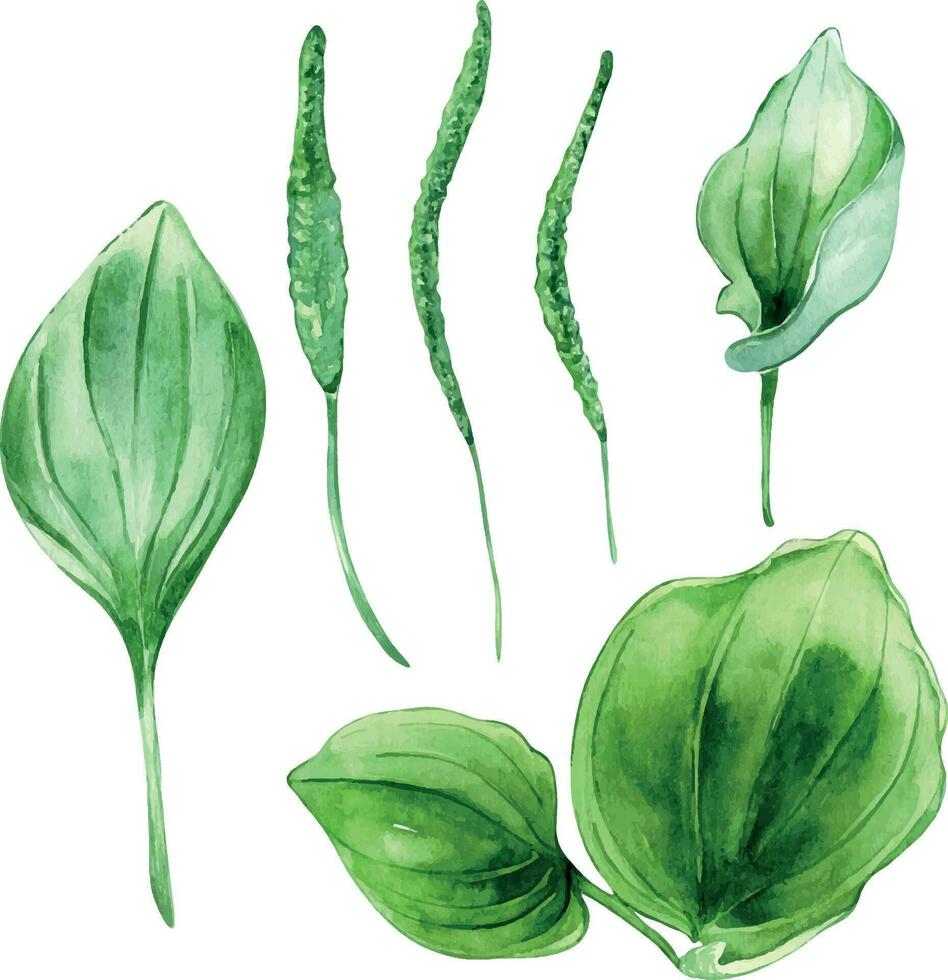The image is a detailed drawing, possibly created with watercolors, featuring a variety of green leaves and pods set against a completely white background. There are a total of six green leaves and pods. The composition includes five vertically standing leaves with three narrow, cylindrical, and slightly curved leaves clustered in the upper middle part of the image. On the left side, there is a single teardrop-shaped leaf with a visible stem. In the lower right corner, two overlapping leaves point diagonally to the right and to the left, exhibiting a mix of light and darker green shades that give the foliage a realistic depth. Each leaf and pod is detailed, showing a bumpy texture and suggesting they might contain seeds. This meticulous portrayal captures the different shapes and subtle color variations within the leaves, emphasizing their naturalistic, watercolor style.